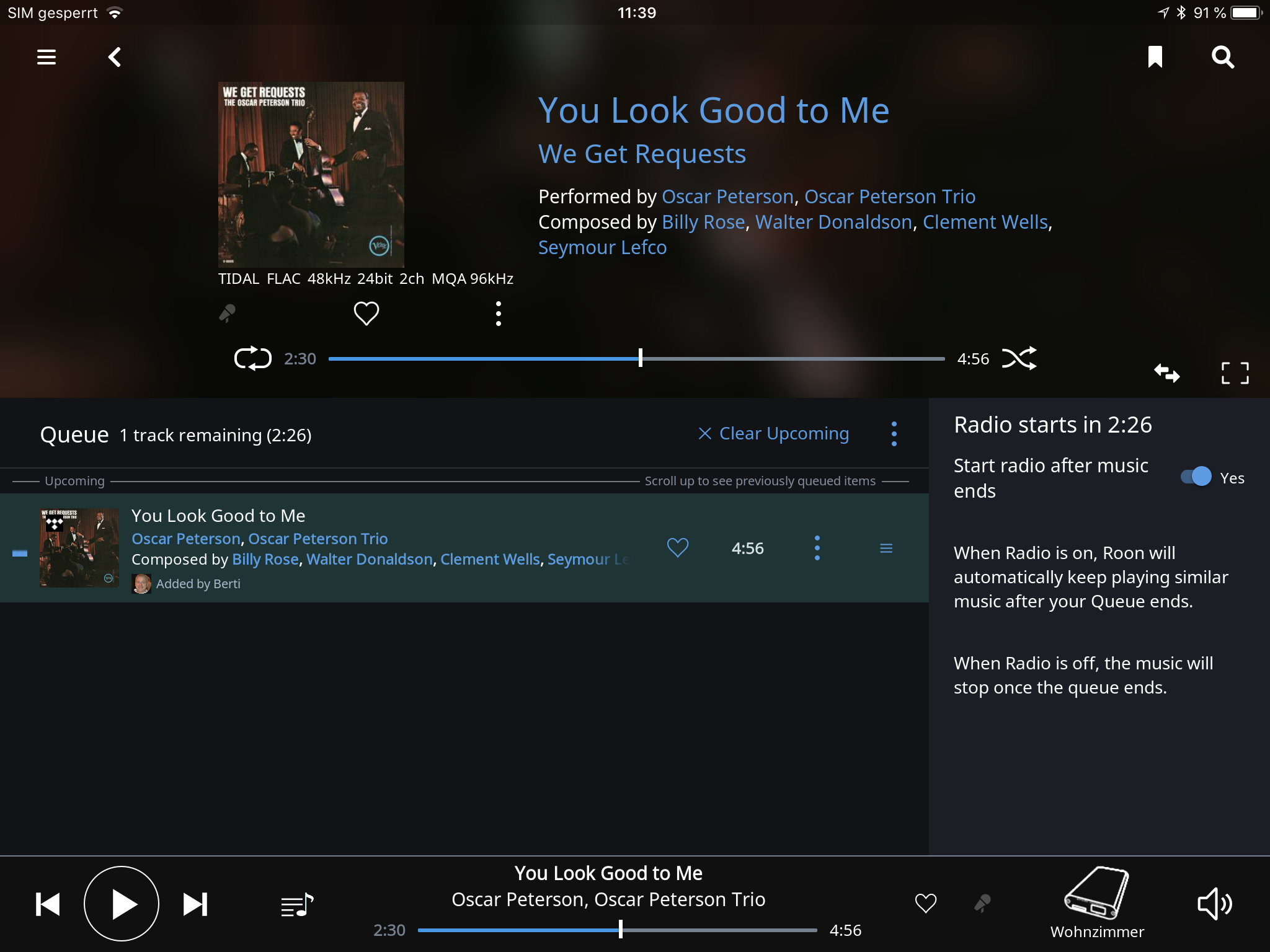The image depicts the screen of an audio player, likely on an Apple device or tablet, as indicated by the Wi-Fi connection status at the top. The currently playing track is "You Look Good to Me" from the album "We Get Requests," performed by the Oscar Peterson Trio. The album artwork on the left side of the screen features three men playing classical instruments.

Details on the screen specify that the song is composed by Billy Rose, Walter Donaldson, Clement Wells, and Seymour Lefkoe. The playback progress shows the track at 2 minutes and 30 seconds out of a total duration of 4 minutes and 56 seconds. Below, the queue indicates one remaining track with a runtime of 2 minutes and 26 seconds. To the right of the queue, there's an option to "Clear Upcoming."

Additionally, the same currently playing song is reiterated in the queue, suggesting it was previously queued. At the bottom left, a notification states "Radio starts in 2.26," with a toggle set to "Yes" for the option "Start radio after music ends." This feature is explained with a note that when the radio is on, the system, likely Rune, will continue playing similar music after the queue finishes.

At the bottom of the screen, standard playback controls for play, fast forward, and rewind are visible.